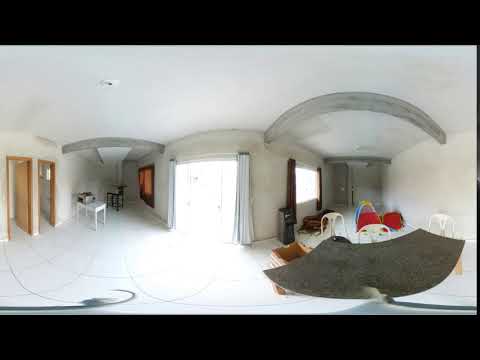This horizontal, rectangular image features a thick black border at the top and bottom, framing a distorted view of a house interior taken with a special lens that curves the perspective. The room is predominantly white, with walls and a floor painted in the same hue, giving a sense of brightness and openness. Straight ahead is a window adorned with gray drapes on either side, allowing natural light to flood the space. To the left, the room extends into a darker area of the house, where a table and two doors leading to other parts of the home are visible. On the right side, an archway opens into another section of the house, featuring furniture including a striking red chair or footstool. This adjacent room also contains a window positioned on a different wall, contributing to the home's airy atmosphere. The curved lens effect gives the ceilings, walls, and certain furnishings like an area rug at the bottom right a bent, rounded appearance, enhancing the image's unique and warped perspective.